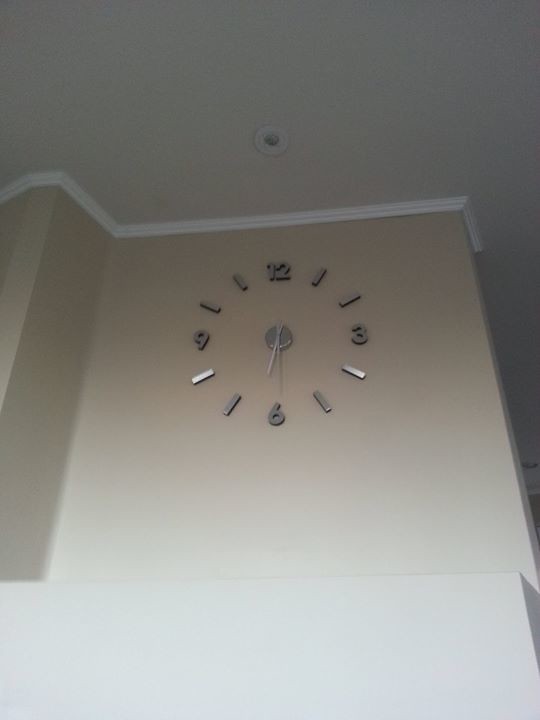This vertical, rectangular color photograph captures a modern wall clock affixed to a cream-colored wall, positioned just below a white ceiling with white molding and a small circular vent. The unique design of the clock omits a traditional frame or border, showcasing only the essential elements. The clock features prominent silver numbers at 12, 3, 6, and 9 positions, while the remaining hours are indicated by slender silver lines, resembling magnets. The clock’s silver hands, including a very thin minute hand, radiate from a central round piece. The time displayed is approximately 6:30.